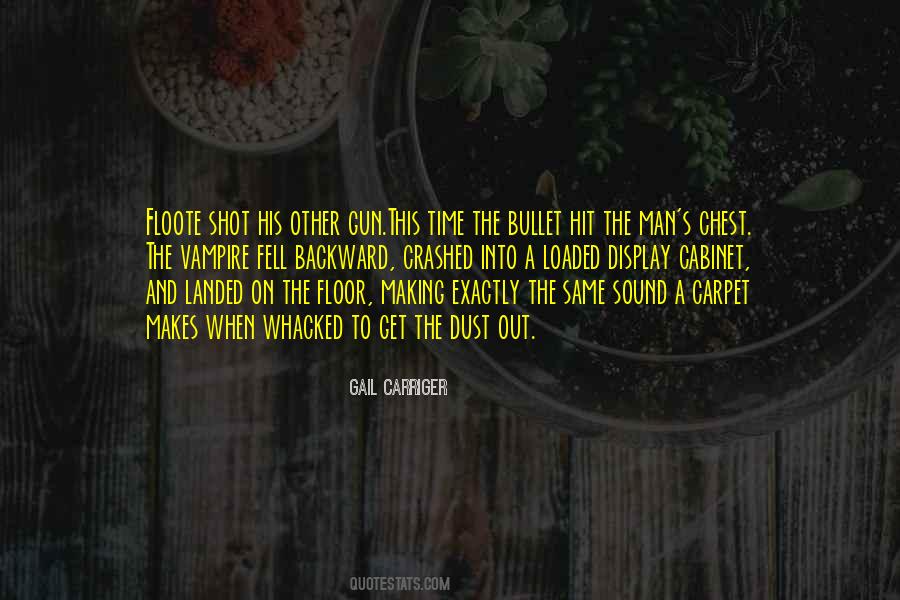The image features an overhead photograph of two planters positioned against a wooden floor backdrop. The planter on the left is white and contains a red or orange cactus with white stones at its base. The right planter is gray and filled with black soil and various small green cactus plants. Positioned in the upper right corner of the image, these planters provide a natural and earthy element to the composition.

Superimposed on the image is a quote in bold yellow capital letters: "FLUTE SHOT HIS OTHER GUN. THIS TIME THE BULLET HIT THE MAN'S CHEST. THE VAMPIRE FELL BACKWARD, CRASHED INTO A LOADED DISPLAY CABINET, AND LANDED ON THE FLOOR, MAKING EXACTLY THE SAME SOUND A CARPET MAKES WHEN WHACKED TO GET THE DUST OUT." Below the quote, in a smaller white font and also in capital letters, it reads: "GAIL CARRIGER - QUOTESTATS.COM." 

This detailed composition combines elements of nature with intriguing textual content, creating a visually and contextually rich image.